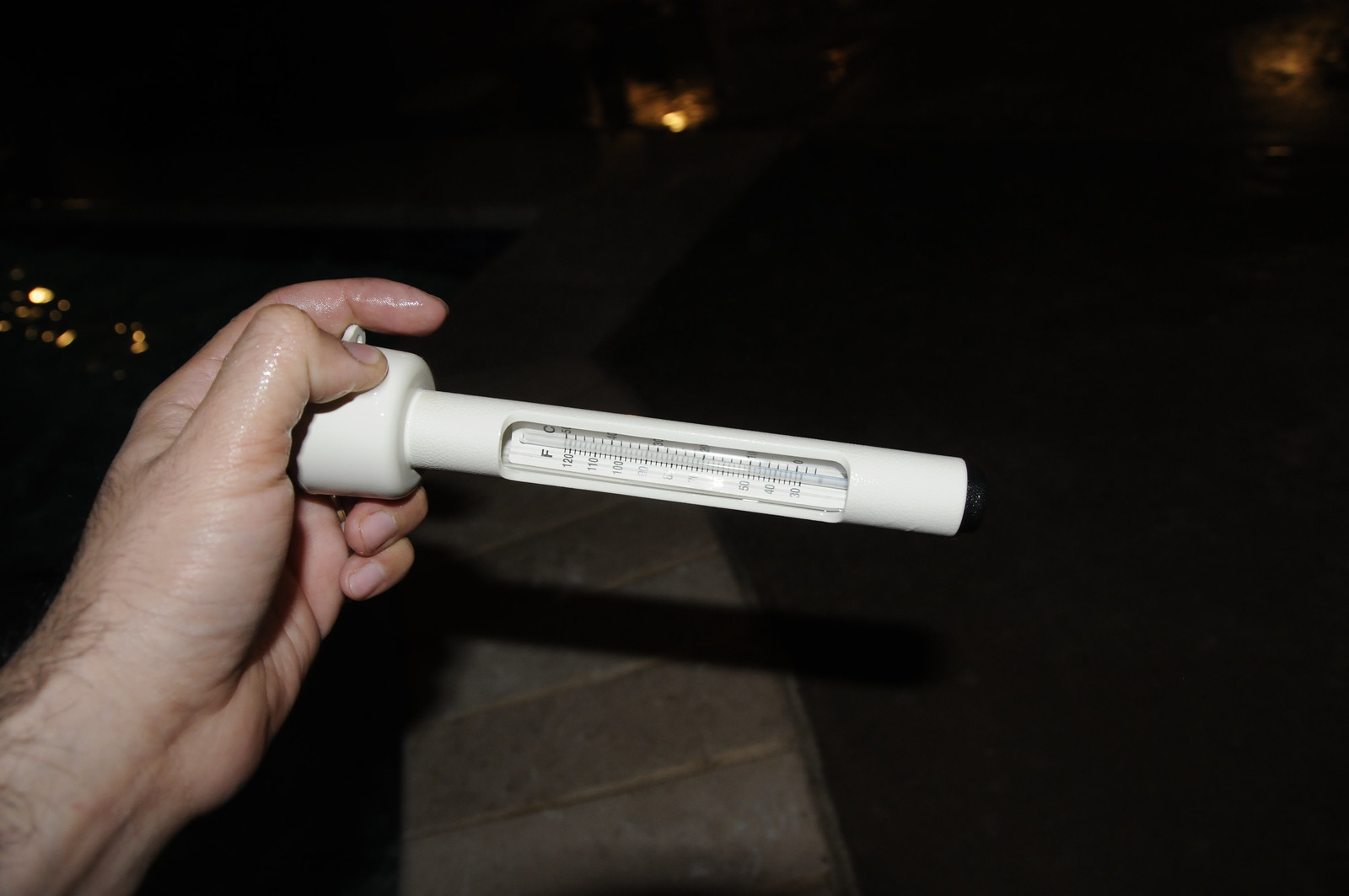In the photograph, a person with a light-skinned, hairy hand is holding up a rod-shaped thermometer. The device is housed in a white, tubular sleeve with a slightly enlarged bottom resembling a small tub, which features a cutout in its center. Through this cutout, the white thermometer is visible, showcasing a glass rod in the middle. The Fahrenheit scale, ranging from 30 to 120 degrees, is situated on the right side, while the Celsius scale is partially obscured on the left, with only the 'C' character visible. 

The scene is set outdoors at nighttime, with the hand illuminated by an external light source, casting a shadow onto a concrete path below. While much of the background is shrouded in darkness, a few distant lights are faintly visible, hinting at an urban or suburban environment.